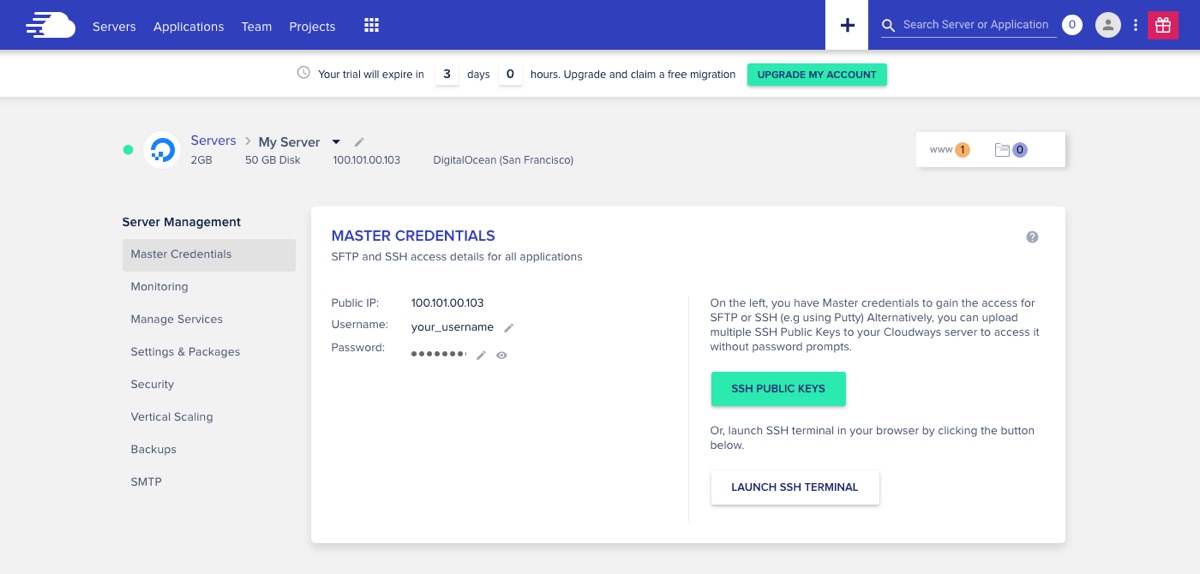Screenshot Description:

The screenshot displays a web interface with a blue banner running across the top. On the left side of the banner, there is a white cloud icon followed by white text reading "Servers," "Applications," "Teams," and "Projects." Next to these, there is a white box with a plus sign inside it. Toward the right side of the banner, there is a search field labeled "Search server or application."

Below the banner, in distinct blue and gray text, the section is labeled "Servers." The information reads "My Server," detailing specifications such as "2 GB," "50 GB Disk," with an IP address "100.101.100.103" repeated twice. The server is associated with "DigitalOcean" and is located in "San Francisco."

Further down, within a rectangular box, blue text labeled "Master Credentials" is displayed prominently. The gray text below it provides details about "SFTP and SSH access details for the applications." Specifically, it notes the "Public IP: 100.101.00.103." 

On the right side of the box, there is a descriptor section explaining that on the left, master credentials can be used to gain access via SFTP or SSH. It also mentions that users can upload multiple SSH public keys to the Cloudways server to bypass password prompts for easier access.